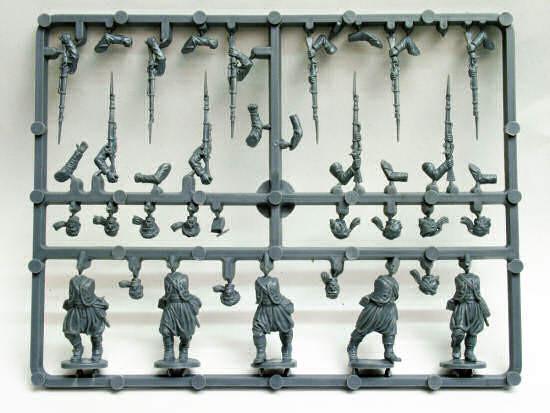This image showcases a gray, plastic frame from a model-making kit, specifically army-themed. At the bottom, the frame holds five human figurines with their heads detached and placed nearby. Above the figurines, there are various accessories intended to be assembled with the model, including multiple arms equipped with large rifles. The plastic frame features two vertical and one central horizontal support, organizing the components for easy snapping off. The entire piece, bathed in muted dark gray color, is positioned on a white backdrop, with shadows casting behind it, adding depth to the scene. The photograph does not include any text or real-life individuals, focusing purely on the detailed model kit components.